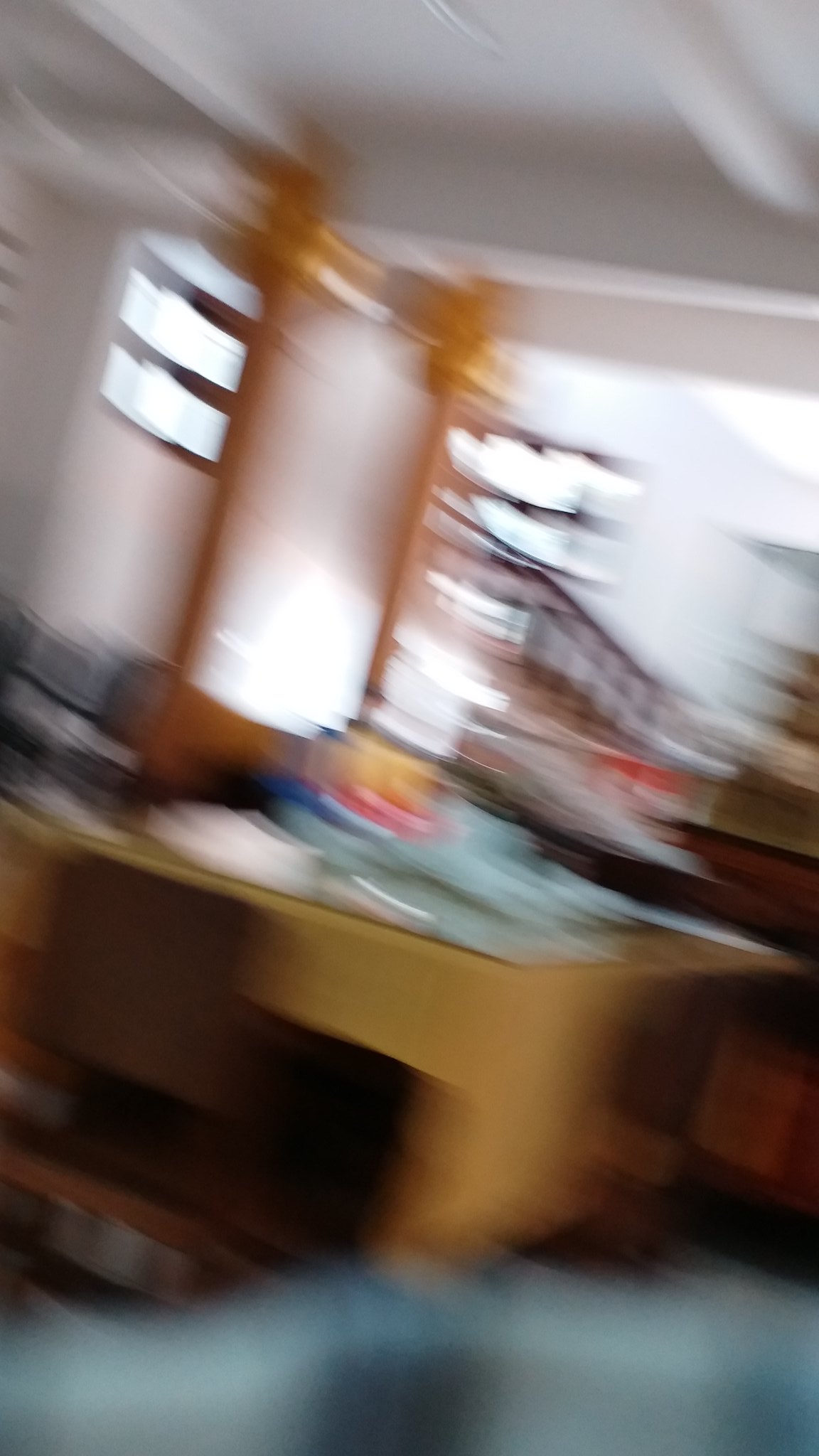This photo, taken in portrait mode on a phone, depicts a chaotic interior scene captured in a rush, resulting in significant blurriness. Central to the image is a large, sturdy wooden desk cluttered with various objects, possibly study materials, hinting at either a study or library setting. Behind the desk, a taller piece of furniture, somewhat resembling a vanity or mirror, adds to the confusion. The background reveals a staircase with a brown banister leading upward, flanked by white walls and windows. On the left side of the image, a sofa or possibly a pool table pushed against the wall can be faintly discerned. Also present are faint outlines of cardboard boxes, suggesting a state of transition or moving. Overall, the frantic nature of the shot makes it challenging to definitively identify all elements, but the scene is filled with a blend of domestic and potentially study-related items.